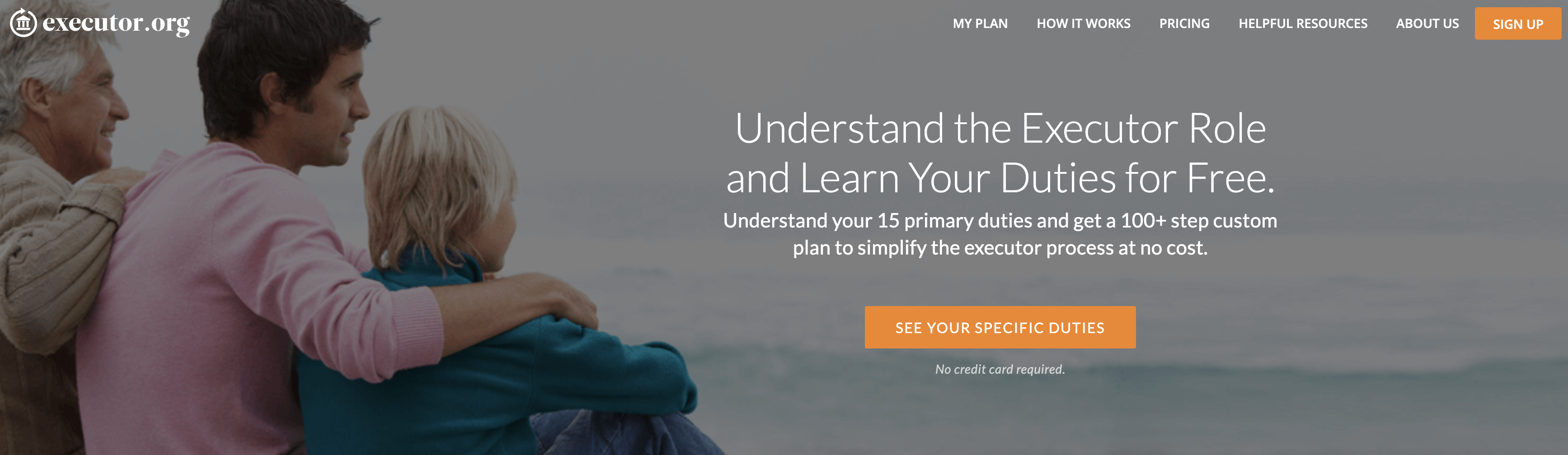This screenshot features an advertisement from executor.org, utilizing a stock photo as its background. The image depicts three generations of a family, with a grandfather placing his arm over his son, who in turn has his arm around his grandson. They stand together, gazing into the distance, and the photograph is taken from behind, showing only the backs of their heads.

Overlaying the image, the text at the top reads "executor.org." Below, a prominent message states, "Understand the Executor Role and Learn Your Duties for Free." Additional text invites viewers to "Understand your 15 primary duties and get a 100+ step custom plan to simplify the executor process at no cost." Below this, there's an orange button labeled "See Your Specific Duties," followed by a reassuring note: "No credit card required."

In the upper right corner of the screenshot, there are several navigation options: "My Plan," "How It Works," "Pricing," "Helpful Resources," and "About Us," although the presence of a "Pricing" tab is somewhat contradictory given the emphasis on the free service.